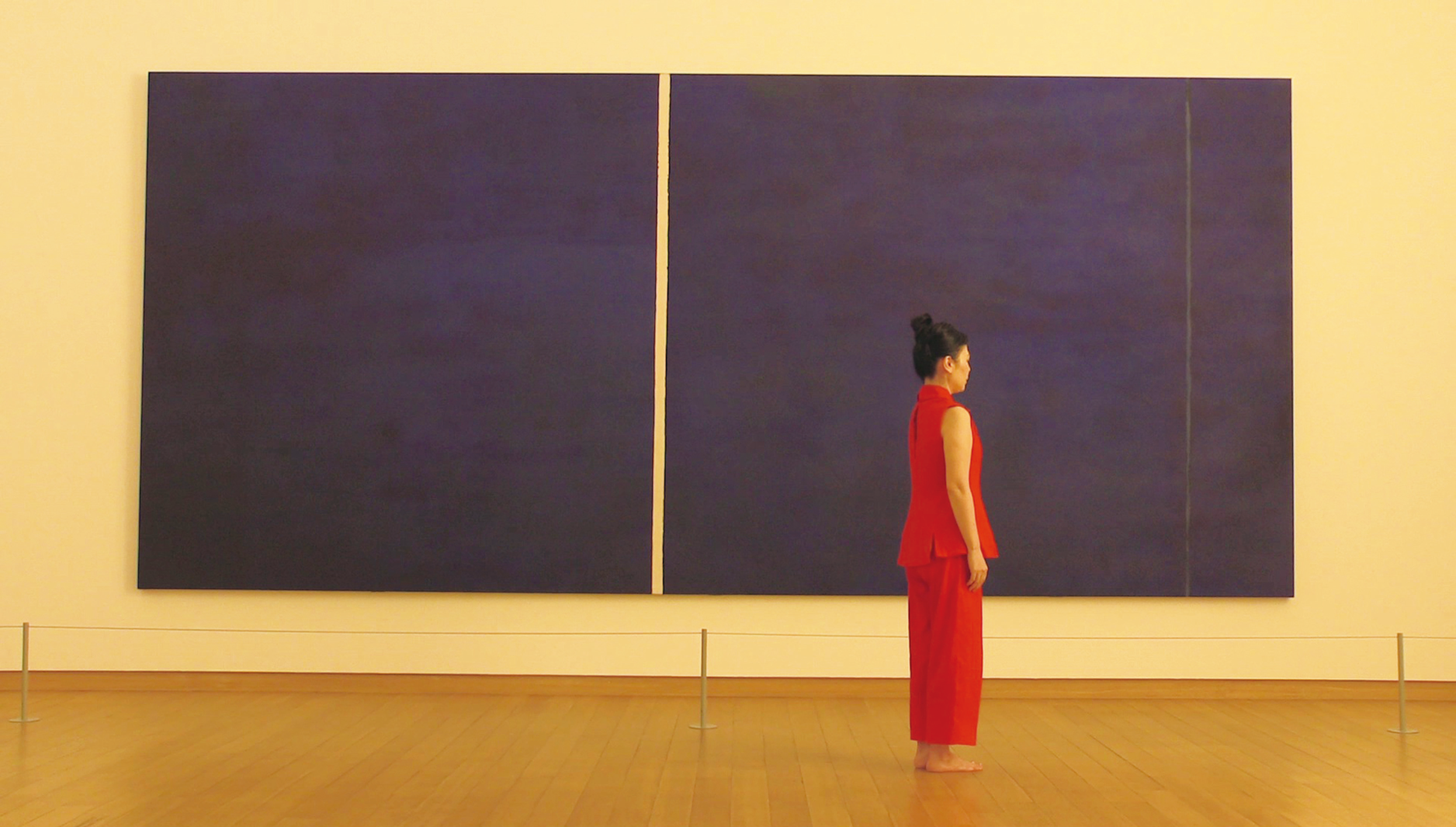This photograph was taken inside a museum featuring a warm, yellowish-tinted wall and an orangish wooden floor. Dominating the wall is a large, split-panel painting comprising two sections: one square and one rectangle, both in a deep blue hue with swirling textures. The square section has a mix of muted colors blending into the blue, while the rectangular piece is marked by a fine, yellowish line running vertically from top to bottom. In front of the painting stands a Japanese woman in a red pantsuit with bare feet. She has her dark hair tied up in a bun and is standing stiffly with her arms at her sides, facing slightly to the right. Her fair to tan skin contrasts with the vibrant outfit. A rope barrier supported by three small pillars is placed in front to prevent viewers from approaching too close to the artwork.